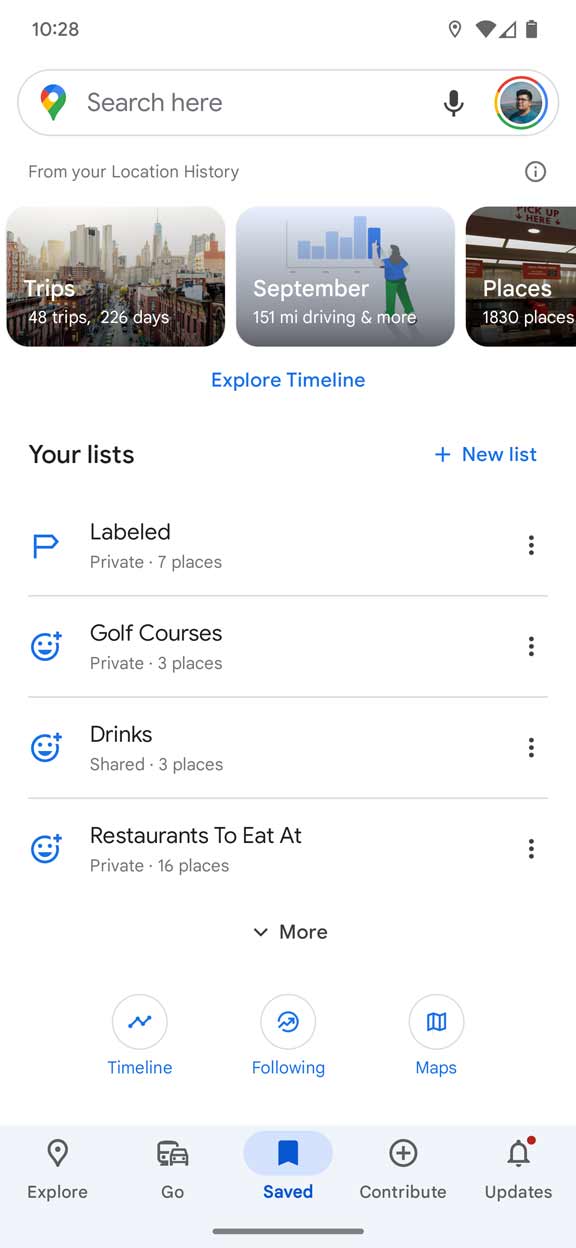A Google search page is displayed, showcasing a user's settings at the top. The search bar clearly shows the user's profile picture within a small, round Google icon adorned with the characteristic rainbow colors. Below the search bar, categories such as "Trips," "September and Places," "Explore Timeline," and "Your Lists" are visible. The user has meticulously added seven places to his list, labeled three golf courses, three places for drinks, and sixteen restaurants. A "More" option is available for further exploration.

Beneath these sections, three circular options labeled "Timeline," "Following," and "Maps" are presented in blue text. The entire interface is set against a white background with predominantly black and blue text for clarity. At the bottom, a navigation bar includes options for "Explore," "Go," "Saved," "Contribute," and "Updates." The "Saved" option is currently selected, and a red dot indicates that the "Updates" section likely has pending notifications or app updates requiring the user's attention.